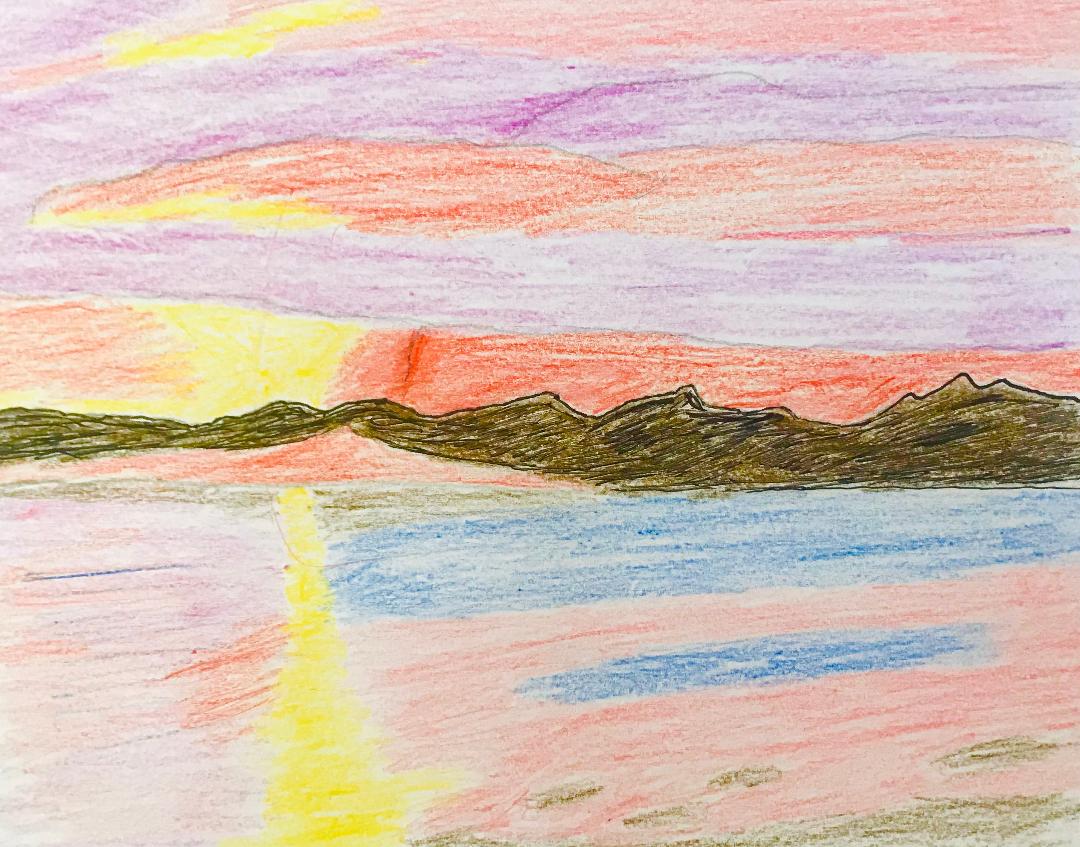This image depicts a childlike drawing of a vibrant and imaginative landscape, rendered in bright, varied colors using either crayons or pencils. Dominating the horizon are dark brown mountains with hues of orange and pink lying above them. The sky transitions through bands of purple, yellow, and orange, encompassing both more concentrated and shaded patches, indicative of a setting sun. The sun itself is portrayed as a bright yellow streak on the left side, casting its light downward.

Moving down the image, the landscape unfolds with a body of water that displays a fascinating mix of colors. On the right side, the water appears blue, transitioning to a pinkish white hue on the left. Intriguingly, there's a pink stretch extending from the sky down towards the hills and further down the page, intersected sporadically by patches of brown and blue.

At the base of this composition, elements resembling land or sandy areas are evident, combining shades of blue, light orange, and additional brown patches. Overall, the drawing is a playful and expressive piece, blending vibrant yellows, purples, and oranges to create a unique interpretation of a natural scene.